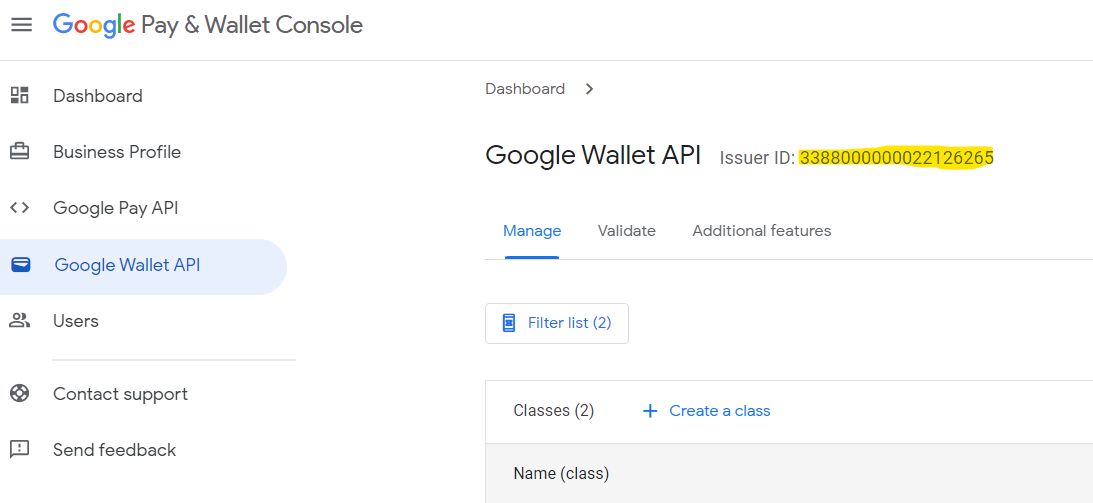The image is a screenshot of the Google Pay website, featuring a predominantly white background with mostly gray text. Some elements are highlighted in blue to draw attention. 

At the top of the screenshot, the text "Google Pay and Wallet Console" is displayed, with "Google" styled in the company's iconic multi-color logo. 

Along the left side of the screen, there's a vertical menu with various clickable headings. From top to bottom, these are:
1. Dashboard
2. Business Profile
3. Google Pay API
4. Google Wallet API
5. Users
6. Contact Support
7. Send Feedback

Currently, the "Google Wallet API" section is selected, signified by its blue text.

On the right side of the screen, the top part features a smaller font text that states "Dashboard." Below this, in a larger font, it says "Google Wallet API issuer ID 338800000000221126265," with the issuer ID number highlighted in yellow. 

Underneath the issuer ID, there are options labeled "Manage," "Validate," and "Additional Features," with "Manage" currently selected, indicated by blue text. Further down, there are additional options - "Filter List 2" and "Classes 2," also in blue font. Adjacent to "Classes 2," there is a clickable plus sign with the label "Create a Class" in blue text.

Overall, the layout clearly delineates various sections and options within the Google Pay and Wallet Console, emphasizing active selections and interactive elements through the use of color highlights.